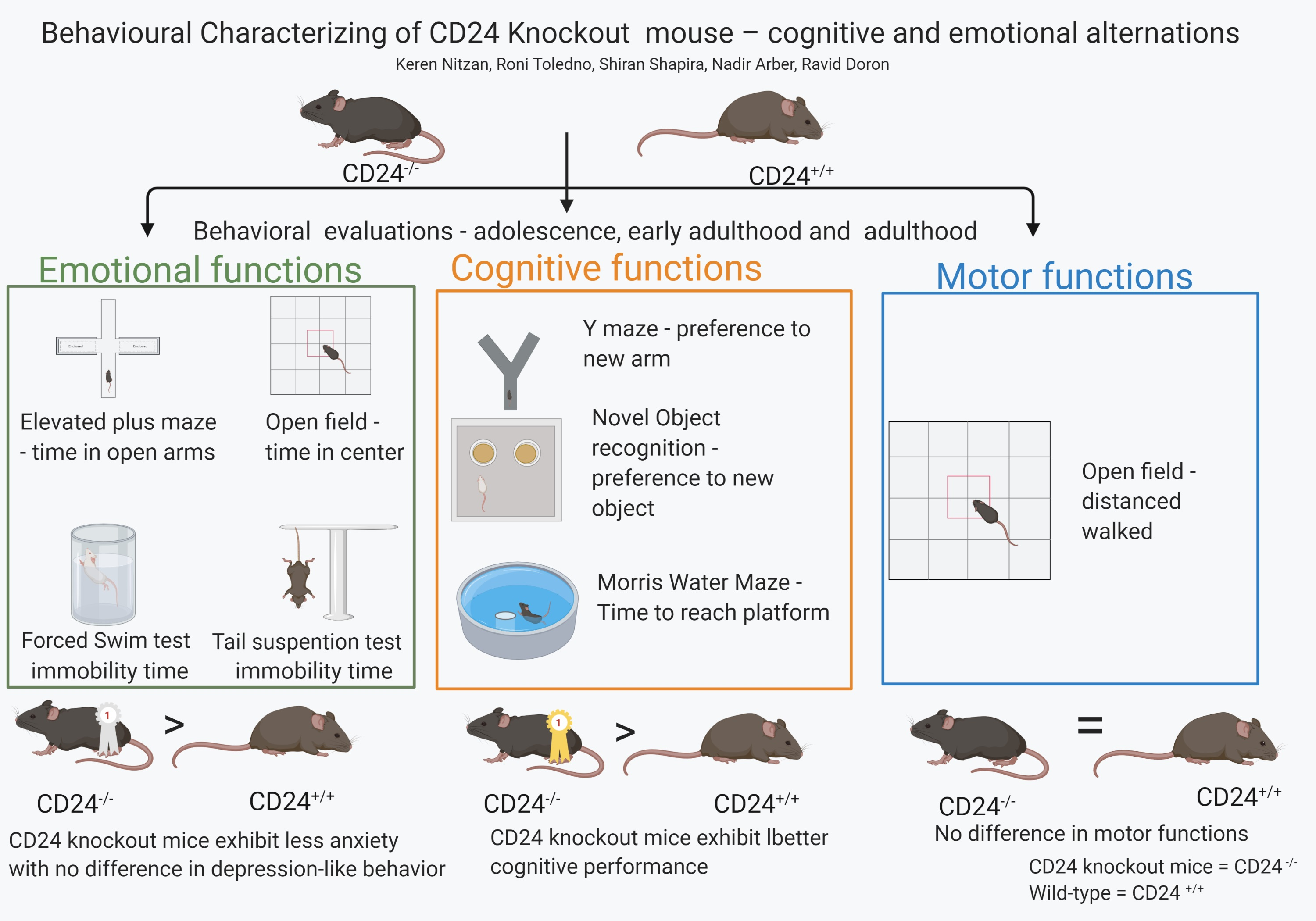The image is a detailed scientific diagram, likely from a textbook or academic paper, titled "Behavioral Characterizing of CD24 Knockout Mouse: Cognitive and Emotional Alterations." It features a horizontally rectangular format with no border and a very light gray background. At the top in black text, the title is prominently displayed, followed by several names.

The diagram includes two main types of brown mice or rats: one labeled "CD24−/−" (dark gray and facing left), and the other labeled "CD24++" (medium gray and facing right). These labels represent different genetic conditions of the mice.

Underneath the mice, there are arrows leading to three categories labeled in colored boxes: "Emotional Functions" (green), "Cognitive Functions" (orange), and "Motor Functions" (blue). Each category contains illustrations of activities the rats might perform, such as treading water or navigating a Y-maze with a preference for one arm.

At the bottom, the diagram features six more rats, each labeled "CD24" along with some having additional symbols or decorations, like a yellow watch. These bottom images include small sentences explaining different behavioral evaluations across life stages: adolescence, early adulthood, and adulthood. Notably, a first-place ribbon indicates that "CD24−/−" mice won in two categories, suggesting superior performance in certain functions.